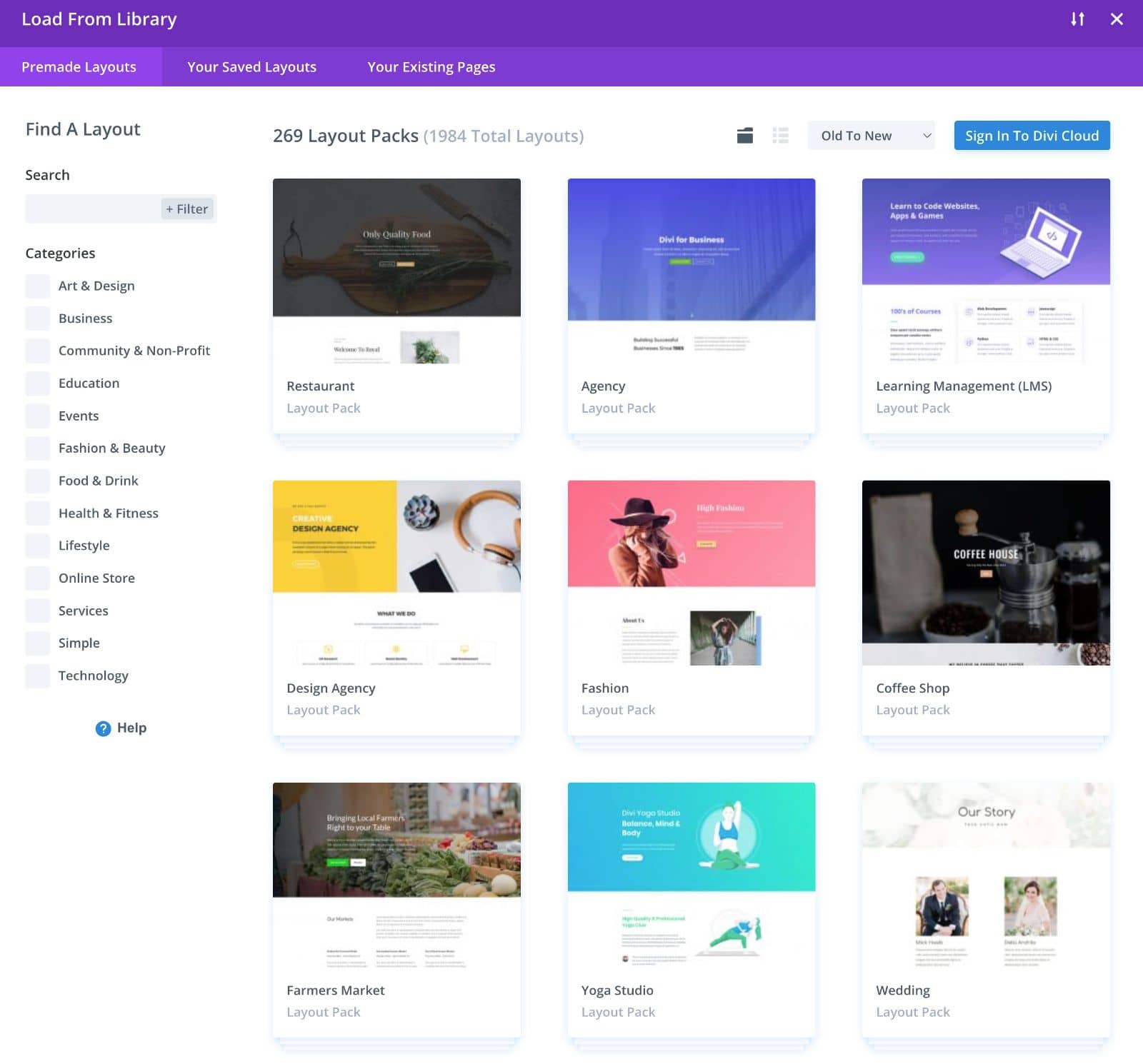The webpage interface is designed with a deep, dark purple header featuring a "Load from Library" button, alongside up-and-down arrows on the right and an 'X' for closing. Below this, in a slightly lighter purple section, are the tabs for "Pre-made Layouts," "Your Saved Layouts," and "Your Existing Pages," with the "Pre-made Layouts" tab highlighted. Against a white background, the top of the page displays the text "Find a Layout" in bold black lettering. Below this, it indicates "269 Layout Packs" and "1984 Total Layouts" in gray parentheses.

There are sorting options labeled "Old" and "New" to arrange the layouts, along with a blue "Sign in to Divi Cloud" link. On the left side, a search bar is provided, accompanied by filter options underneath. The categories listed include: Art and Design, Business, Community and Non-Profit, Education, Events, Fashion and Beauty, Food and Drink, Health and Fitness, Lifestyle, Online Store, Services, Simple, Technology, and a Help button.

Nine layout examples are showcased across the page. These include a black-and-gray restaurant layout (featuring what looks like a pan in the background), a purple agency layout, a layout for learning management that is purple on top and white on the bottom, a yellow design agency layout, a pink fashion layout, and additional layouts for a coffee shop, farmers market, yoga studio, and other pre-made examples for various uses.